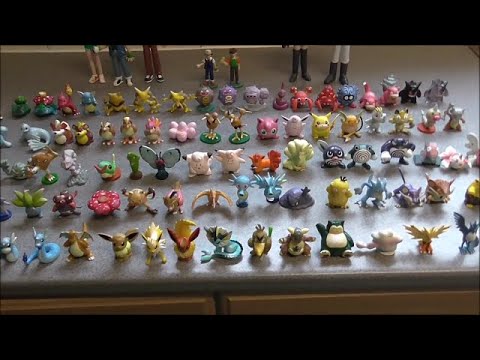In this photograph, a meticulously arranged display of Pokemon figurines can be seen lined up in five distinct rows set on a large, light grey stone-finished countertop or desk. The setup is framed by a wooden shelf above, exhibiting a rich brown tint underneath and a lighter brown top. The collection comprises a diverse array of vibrant, colorful models, including well-known characters such as Snorlax, Eevee, and Psyduck. While the exact number of figurines is unclear, estimates suggest there could be between 60 to 80. Positioned behind these rows are miniature human figurines, visible from the waist down, seemingly observing the Pokemon. These human figures are organized into groups: two shorter figures, presumably children, are centrally located, with three taller figures on the left and two on the right, likely representing adults. Despite the less-than-perfect lighting and image quality, the scene captures a detailed and expansive assembly, reflecting a full generation of the iconic Pokemon universe.